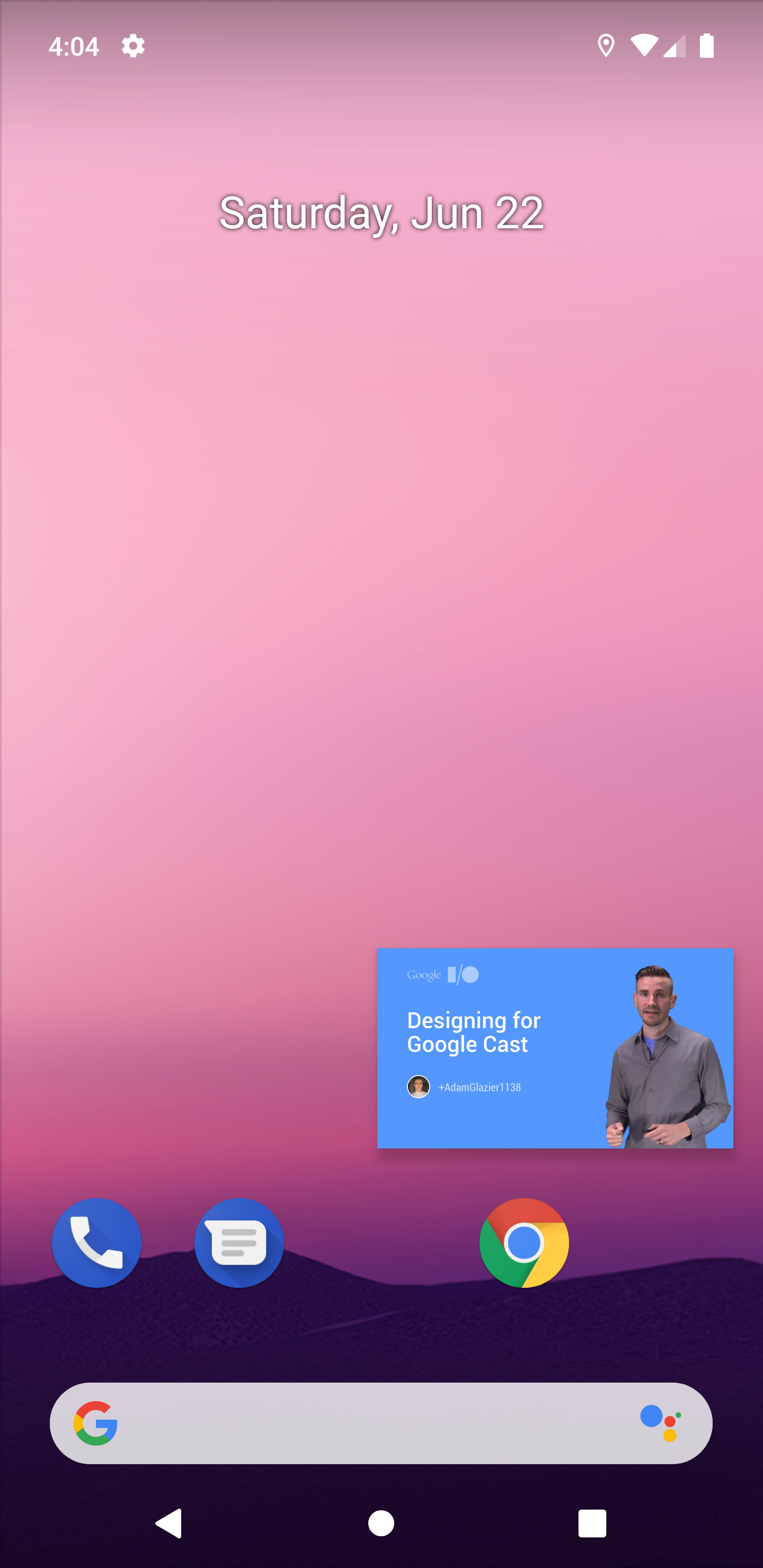The image serves as the background for a mobile device's home screen. In the top-left corner, white numerals display the time reading "4:04," though it's unclear whether it is a.m. or p.m. To the right of the time, a white gear symbol represents the settings icon. Additional icons line up on the far right side of the status bar, including symbols for location, Wi-Fi signal, cellular signal, and battery life.

The background of the home screen exhibits a gradient transitioning from pale pink and bright pink to a blend of purple and hot pink near the bottom. At the very base of the image, mountains provide a scenic touch.

Centrally placed is a widget entitled "Designing for Google Cast," featuring an image of a man. Positioned at the bottom of the screen are icons for essential apps: Phone, Text, and Google Chrome, alongside a search bar.